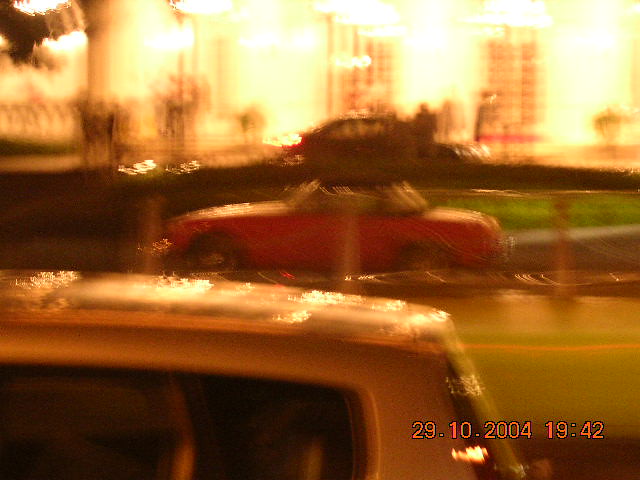A blurry image of a road taken on October 29th, 2004 at 7:42 PM, as indicated by the red timestamp in the bottom right-hand corner of the photograph. The entire image has a slight yellowish tint, possibly due to lighting conditions. 

In the bottom left-hand corner, and predominantly in the focus of the picture, is the roof of a sedan. Just behind it, further down the road, is a small red sports car, though the make and model of both vehicles are indiscernible due to the blurriness. Separating these two cars on the road appears to be a glass wall.

Further back in the image, behind the red car, there is another vehicle and what seems to be two people sitting next to it. The background features an array of buildings, possibly skyscrapers, adding an urban ambiance to the scene.